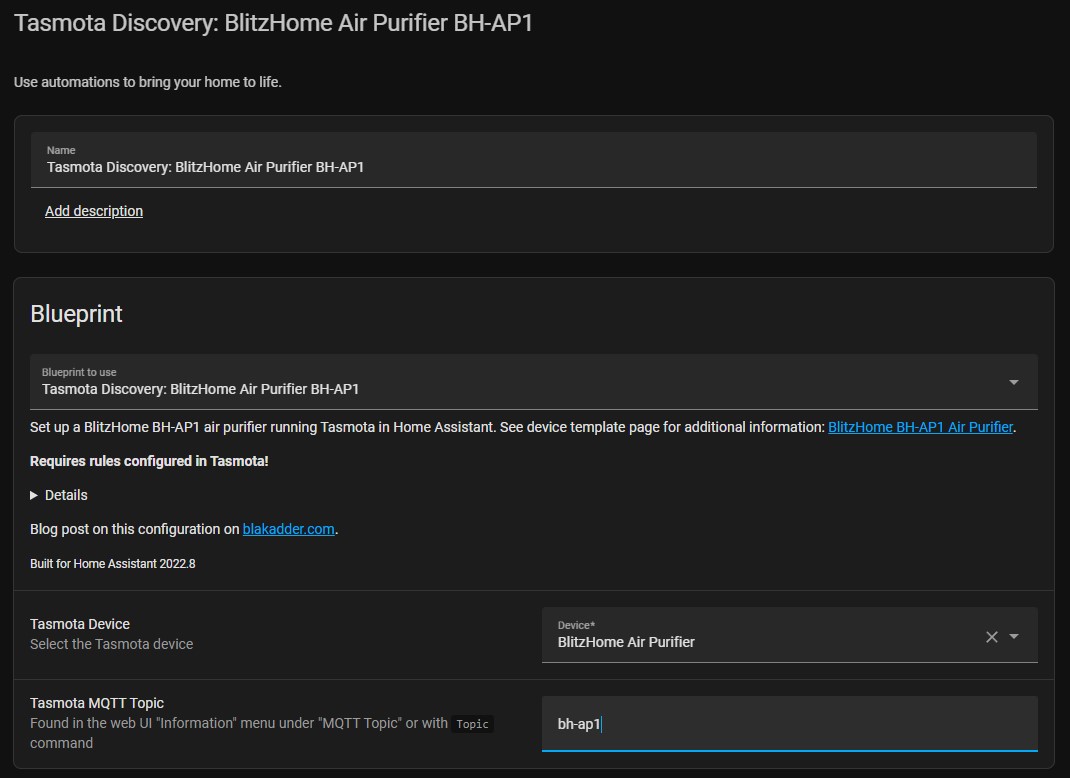Image Description:

The image features a black background with white text prominently displayed at the top. The main headline reads "Tad Motor Discovery" followed by "Blitz Home Air Purifier BHA P1: Use automation to bring your home to life." 

Below this, there is a gray box containing text that repeats the headline: "Tad Motor Discovery Blitz Home Air Purifier BHA P1." Underneath this box, the text reads "Add Description" followed by another line that says "Blueprint."

A second gray box is situated beneath, repeating the phrase "Blueprint to use Tad Motor Discovery Blitz Home Air Purifier BHA P1." Below the second gray box, detailed instructional text is provided: "Set up a Blitz Home BHA P1 air purifier running Tad Motor and Home Assistant. See device template page for additional information. Requires rules configured in Tad Motor. Details, blog post on this configuration at blackadder.com. Built for Home Assistant 2022 Tad Motor device, select the Tad Motor device."

This detailed caption aims to provide users with comprehensive instructions and additional resources regarding the integration and setup of the Blitz Home Air Purifier BHA P1 with Tad Motor and Home Assistant.